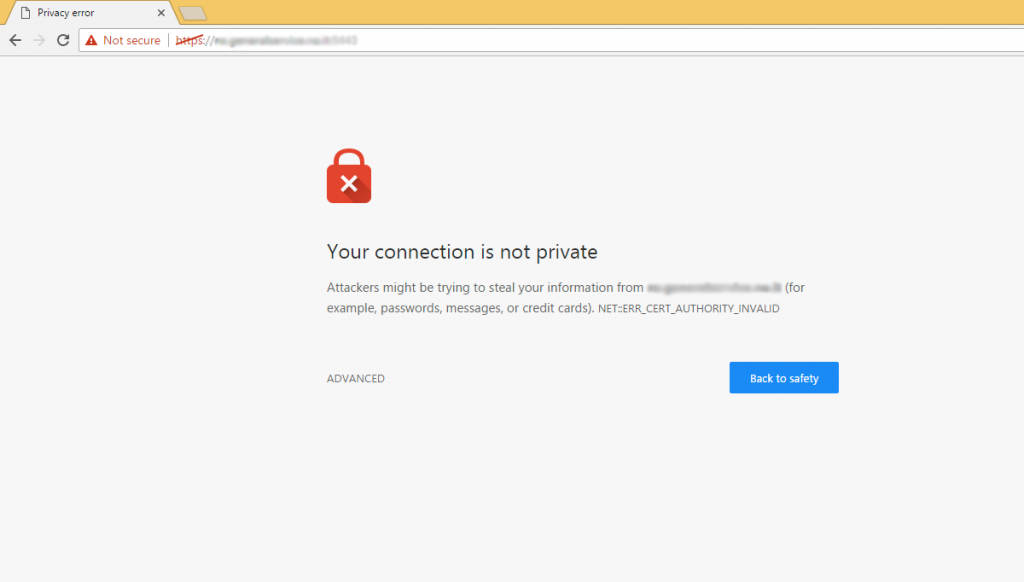The image is a detailed screenshot from a web browser on a computer, illustrating a privacy error. At the very top of the browser, there is a prominent yellow bar indicating an alert. Within this bar is an open tab featuring a small file icon and the text "Privacy Error," with an "X" symbol to the right for closing the tab.

Directly below the yellow bar is the address bar. On the left side of the address bar, a red caution symbol is displayed, accompanied by the text "Not Secure." Next to this, the letters "HTTPS" appear in red with a diagonal strike-through line, indicating an issue with the secure connection. The remainder of the web address is shown in black but is blurred out for privacy.

To the left of the address bar, several navigation buttons are visible: a circular arrow symbolizing the refresh option, a grayed-out forward button, and a standard back button.

The main body of the page displays a large red lock symbol with a white "X" on it, reinforcing the security warning. Below this symbol, bold text states, "Your connection is not private," followed by an explanation: "Attackers may be trying to steal your information from the [blurred web address], for example, passwords, messages, or credit cards."

An error message below this warning reads, "NET::ERR_CERT_AUTHORITY_INVALID," indicating a certificate validation issue. At the bottom of the page, there are two clickable options: a blue button labeled "Back to safety" in white text and a smaller "Advanced" text link to the left of the button.